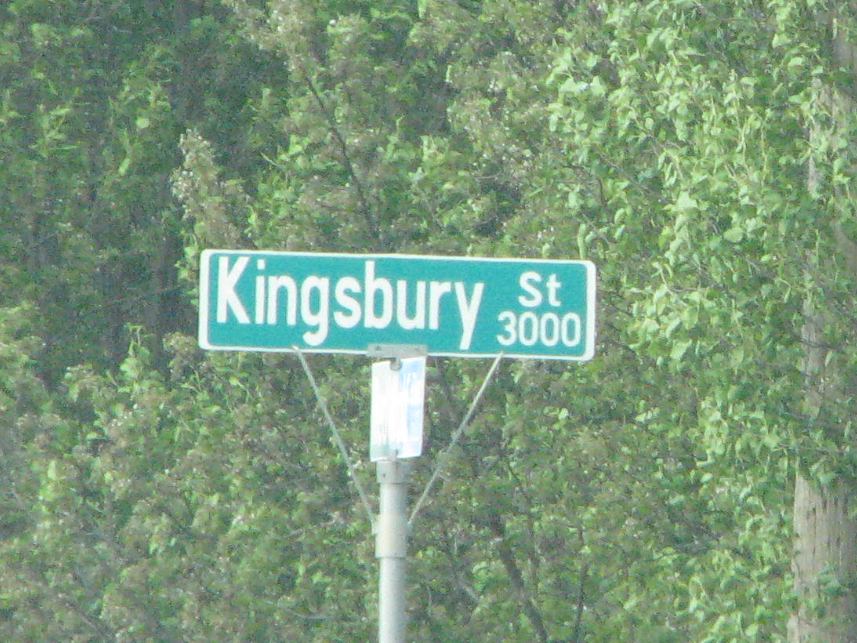The image captures a slightly blurry photograph of a residential street sign surrounded by lush greenery. The sign, primarily dark green with a white border, displays "Kingsbury Street" in large white text, with "Kingsbury" on the left and "ST" above "3000" on the right. Clusters of vibrant green leaves and numerous branches from what seems to be multiple trees dominate the background, with a prominent tree trunk featuring brown bark with dark spots and light stripes visible on the right side. Additionally, a telephone pole is partly visible through the foliage on the right. The street sign is mounted on a steel pole, with another perpendicular sign not fully discernible due to the glare from the sunlight suggesting late afternoon. The overall setting appears to be a wooded residential area, likely during spring or summer, with budding flowers indicative of early growth.